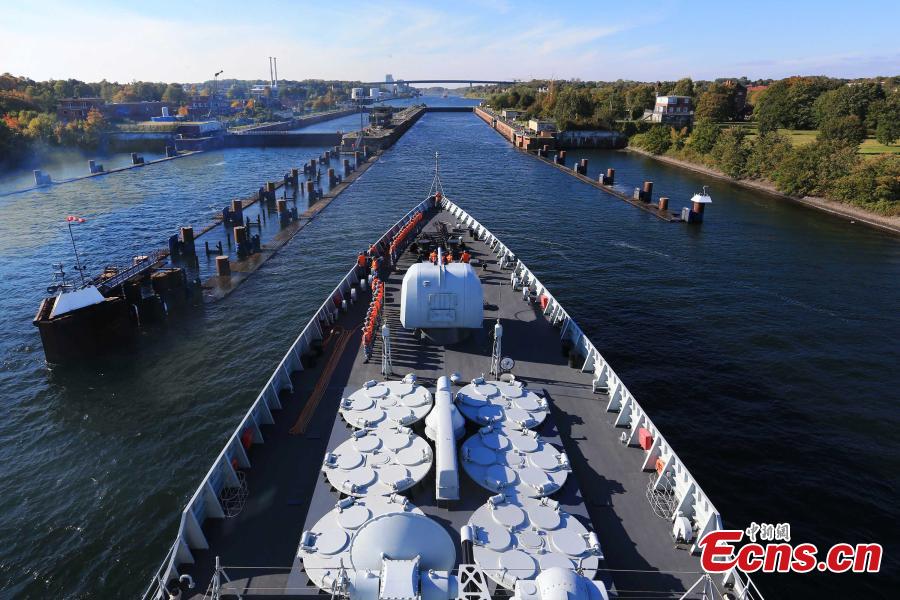The image captures a detailed scene from the deck of a commercial fishing boat, likely a large vessel navigating a wide river maintained by human developments. The photograph, taken from an elevated vantage point such as the captain's office, showcases the forward half of the ship, revealing six large white built-in containers on the deck, each with six holes possibly for storing fish. Various fishing gear in orange, white, and black can be seen towards the front of the boat, although too small to identify precisely. There is a noticeable logo, "ECNS.CN," in red on the bottom right of the image.

In the mid-background, men in gray pants, red shirts, and blue hats stand in a single file line on the port side, indicating structured activity, possibly as the vessel approaches a port. Ahead, a gate, restricting further passage, hints at an upcoming docking procedure. The sides of the river are flanked by trees and scattered small buildings, with some industrial areas visible near the dock. A bridge spans the river, connecting the two sides of the land and suggesting a well-developed infrastructure.

The sky overhead is a mix of white clouds on the left and clear blue on the right, creating a disparate yet harmonious skyscape above the scenic river and busy boat.